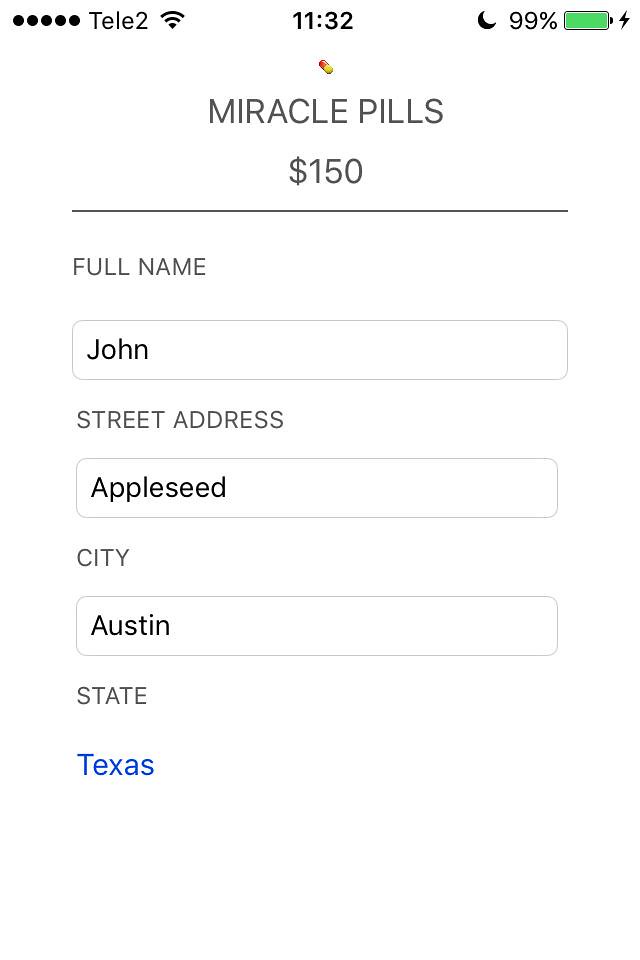The image is a detailed screenshot of a cell phone screen. At the top, it shows the time as 11:32 with Tele 2 service bars on the upper left and a battery icon at 99% with a charging symbol on the upper right. Below, a red and yellow pill icon is prominently displayed, followed by the text "Miracle Pills" in black lettering and a price tag of "$150". A thin horizontal black line separates this section from the form below.

The form fields, which are filled in black text, include:
- Full Name: John
- Street Address: Appleseed
- City: Austin
- State: Texas, printed in blue text

The overall text on the form consists mainly of black and some gray, contributing to a clean and structured layout for the information input.